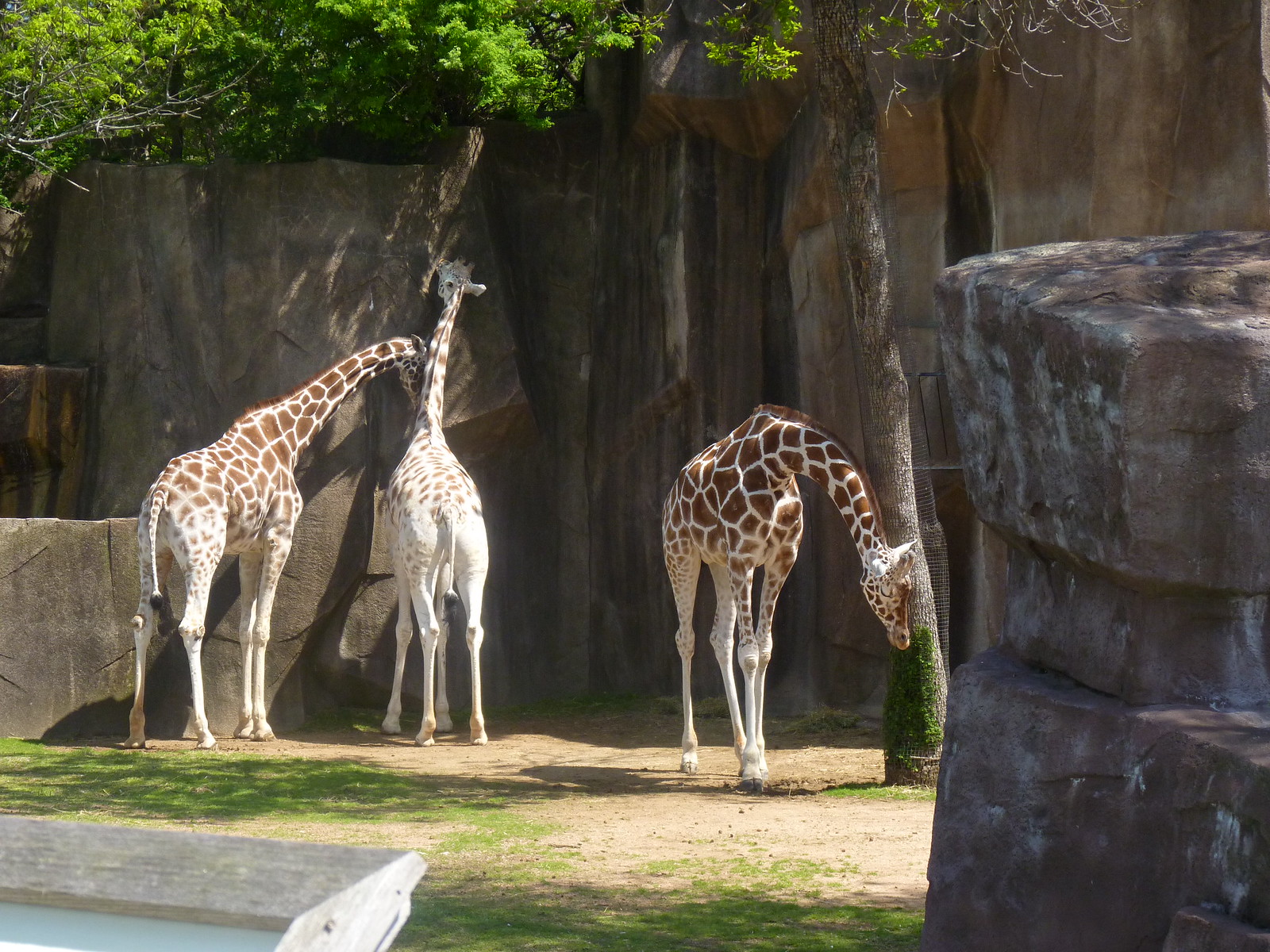This detailed photograph, likely taken at a zoo, showcases three giraffes amidst a zoo-like landscape with tall faux rock walls and vibrant greenery. In the backdrop, two smaller giraffes with intermingling shades of brown and white fur stand closely together by a weathered faux rock formation, seemingly investigating or perhaps napping against it. The giraffe on the left has a darker tone compared to the lighter, sparsely spotted giraffe in the center. Their attention appears diverted, possibly towards the hanging leaves and branches that adorn the top of the rocks. Foregrounded to the right, a solitary giraffe faces the camera but has its head bent down level with its knees, suggesting a resting or grazing posture. This giraffe is framed by a tree slightly behind it, adding depth to the setting. The ground beneath is a mix of dirt and sparse bocce grass, typical of a fabricated habitat, lending authenticity to the scene with a light casting nuanced shadows from the surrounding trees and structures.